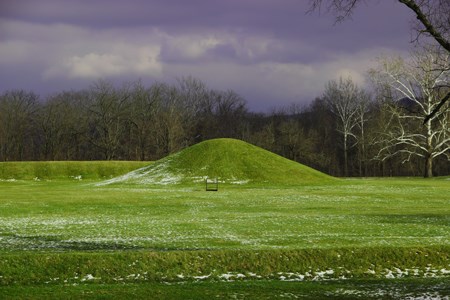The photograph showcases a picturesque nature scene centered around the Hopewell Ceremonial Earthworks, an indigenous mound situated in a wide-open pasture. The large, dome-shaped mound, lush with green grass and lightly dusted with snow on its left side, dominates the foreground. Surrounding the mound is a grassy field, interspersed with patches of white frost, adding a touch of wintry beauty to the landscape. Encircling the field is a dense tree line, predominantly dark green and black, with a striking leafless white birch tree standing out on the right. Above, the sky is overcast, heavy with dark grey and purple clouds, suggesting an imminent rain.